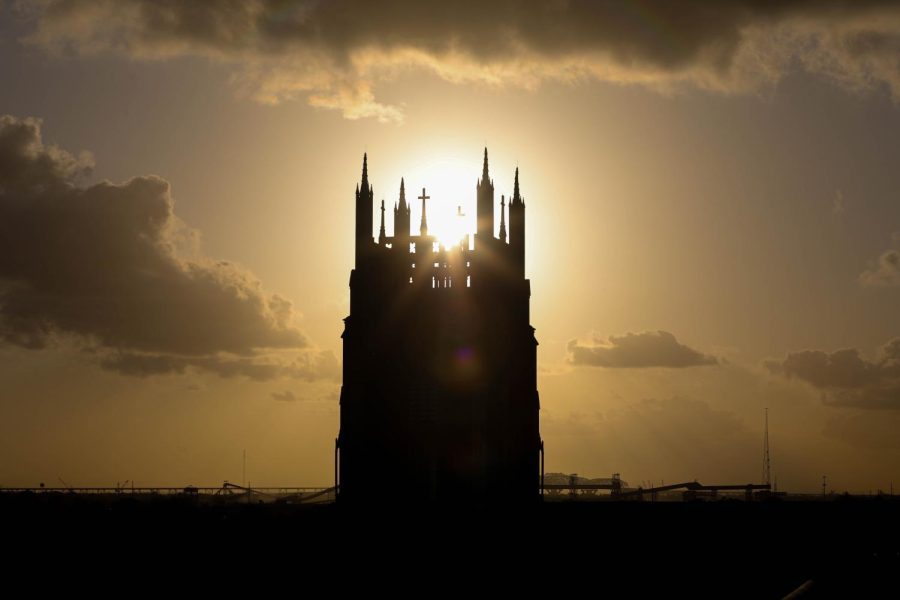This vivid, colored photograph captures a striking scene outdoors, likely during sunset. The heart of the image is a towering church or cathedral structure, prominently featuring a square tower with a cross at its center. At each corner of the tower, a tapering spire rises, creating a dramatic silhouette against the sun, which is positioned directly behind the tower, casting a glowing halo-like effect. The sky is filled with clouds, enhancing the image's majestic atmosphere. In the background, the faint outlines of a cityscape or townscape can be discerned, along with a possible radio or cell phone tower on the right side. The foreground remains almost entirely dark, providing a stark contrast that draws attention upward to the illuminated tower. The overall composition of the image is square, focusing viewers' eyes centrally on the architectural marvel amidst the sky's expanse.